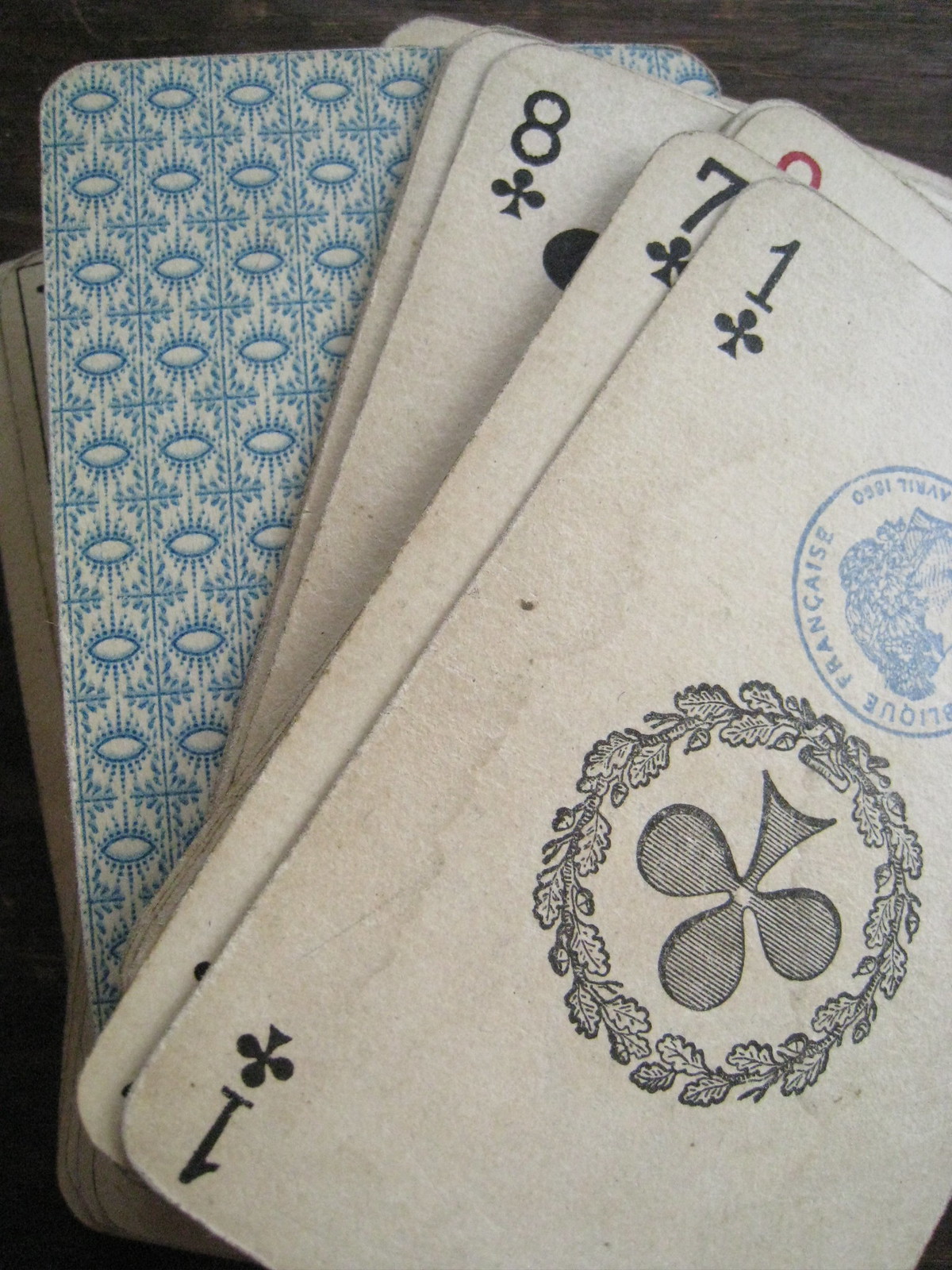In the image, a stack of playing cards is slightly fanned out on a dark wooden table, giving a glimpse of several face-up cards and part of the rest of the deck. At the top of the stack is a seven of clubs, featuring a unique design with an upside-down club symbol surrounded by a circular leaf motif. Additionally, there's a stamp that possibly indicates French origin, as it bears the word "Francois." Seven cards are clearly visible, with intricate club suits, while the eighth card is face-down, displaying a blue patterned back. The edges of a few more cards from the remaining deck peek out beneath, suggesting there are approximately 47 cards in total. A hint of a red number is visible but obscured, adding a touch of mystery to the composition.